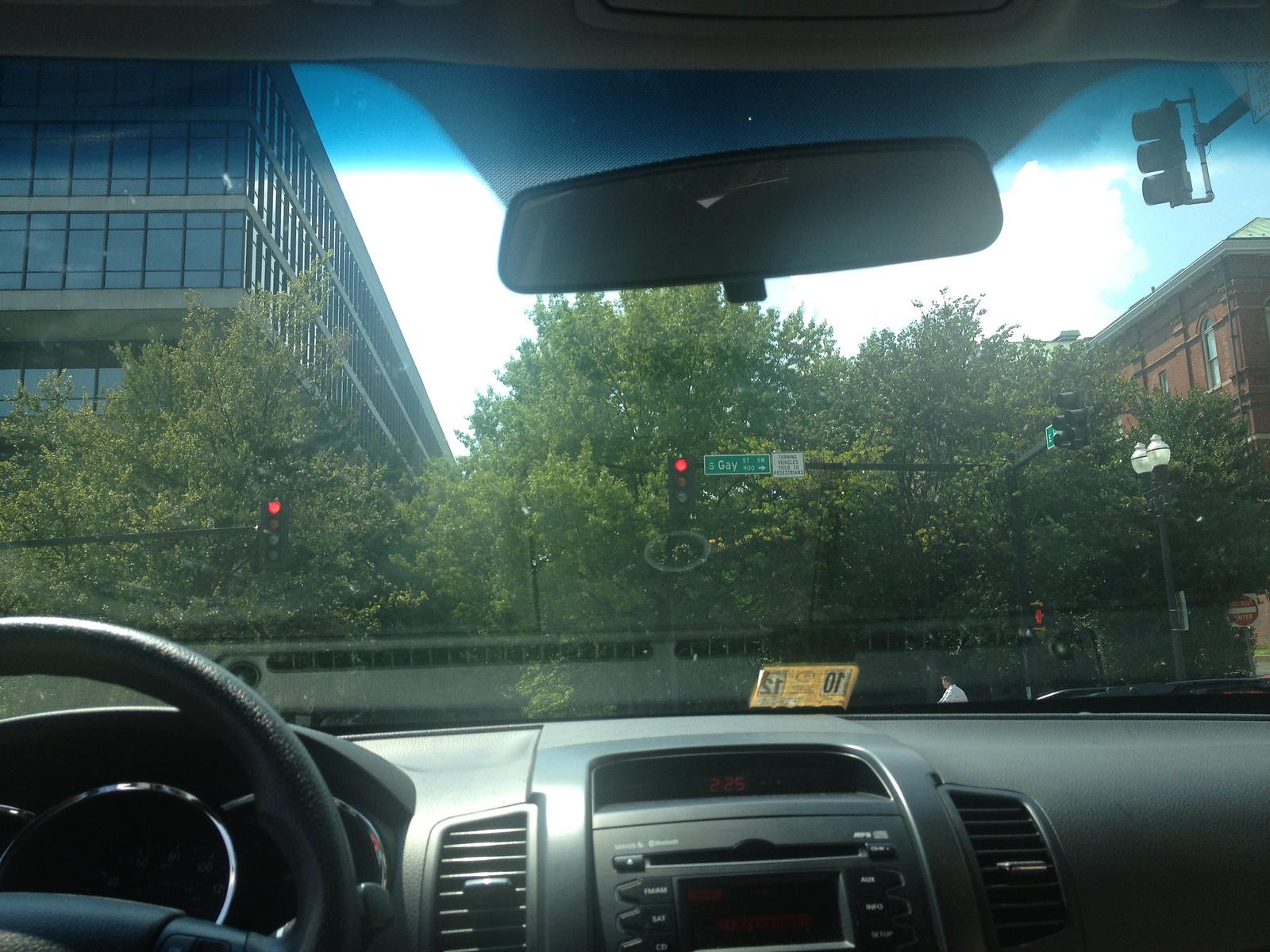The image presents a detailed inside view of a passenger vehicle, taken from the middle of the front seats, possibly by a passenger seated in the back or by automated means. On the lower left, a fragment of the charcoal-colored steering wheel is visible without any hand on it, suggesting the absence of the driver or that the driver is out of frame. The dark gray dashboard displays a digital clock reading 2:25 p.m. in red digits amidst silver-lined speedometers and controls.

The windshield's focal point features a yellow inspection sticker marked "10-12" at its lower center, accompanied by a rearview mirror reflecting the dark-colored back seats. Through the windshield, a red traffic light is clearly illuminated at the intersection of South Gay Street, with another traffic light visible overhead but not clearly indicating its color. The intersection prohibits the driver from proceeding straight ahead.

Ahead, a pedestrian in a white t-shirt is captured from the shoulders up, crossing the street. Surrounding the scene, various landmarks are discernible: to the right, a mix of brick and off-white roofed buildings with light green pitched roofs and structural bars; to the left, a tall glass building. Deciduous trees further enhance the urban backdrop. Additionally, multiple street signs, including a partially obscured one beginning with a 'G' and another small square white sign with black text, contribute to the intricate cityscape visible from the vehicle.